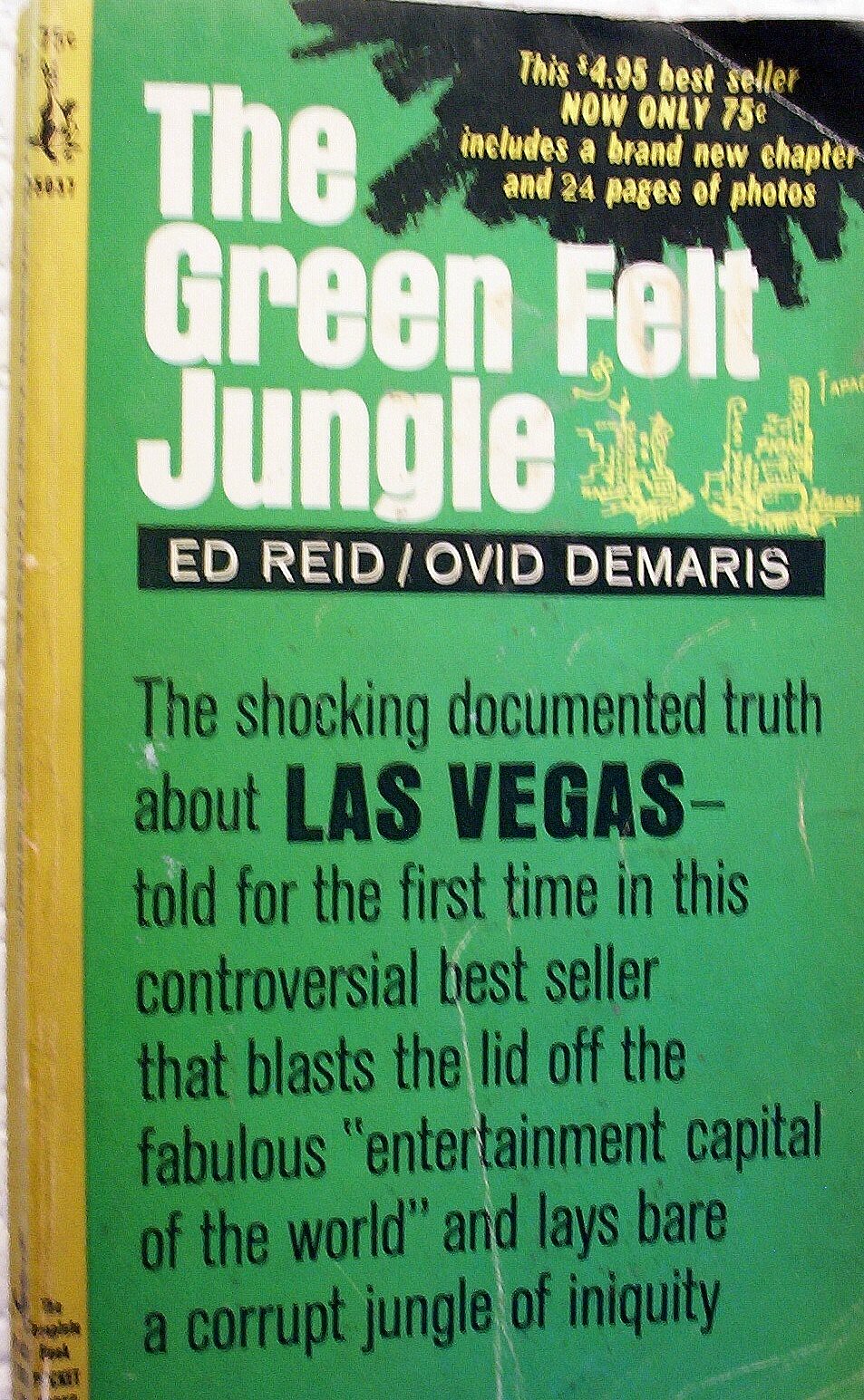The image is a rectangular photograph of a vintage book cover with a green background and a yellow spine. In the upper right-hand corner, there is a splash of black background with yellow text that reads, "This $4.95 bestseller, now only 75 cents, includes a brand new chapter and 24 pages of photos." The book's title is prominently displayed in white font as "The Green Felt Jungle," authored by Ed Reed and Ovid Demaris. Beneath the title, in black text, it declares, "The shocking documented truth about Las Vegas, told for the first time in this controversial bestseller that blasts the lid off the 'fabulous entertainment capital of the world' and lays bare a corrupt jungle of iniquity." The old design and detailed text suggest it is a vintage book cover.